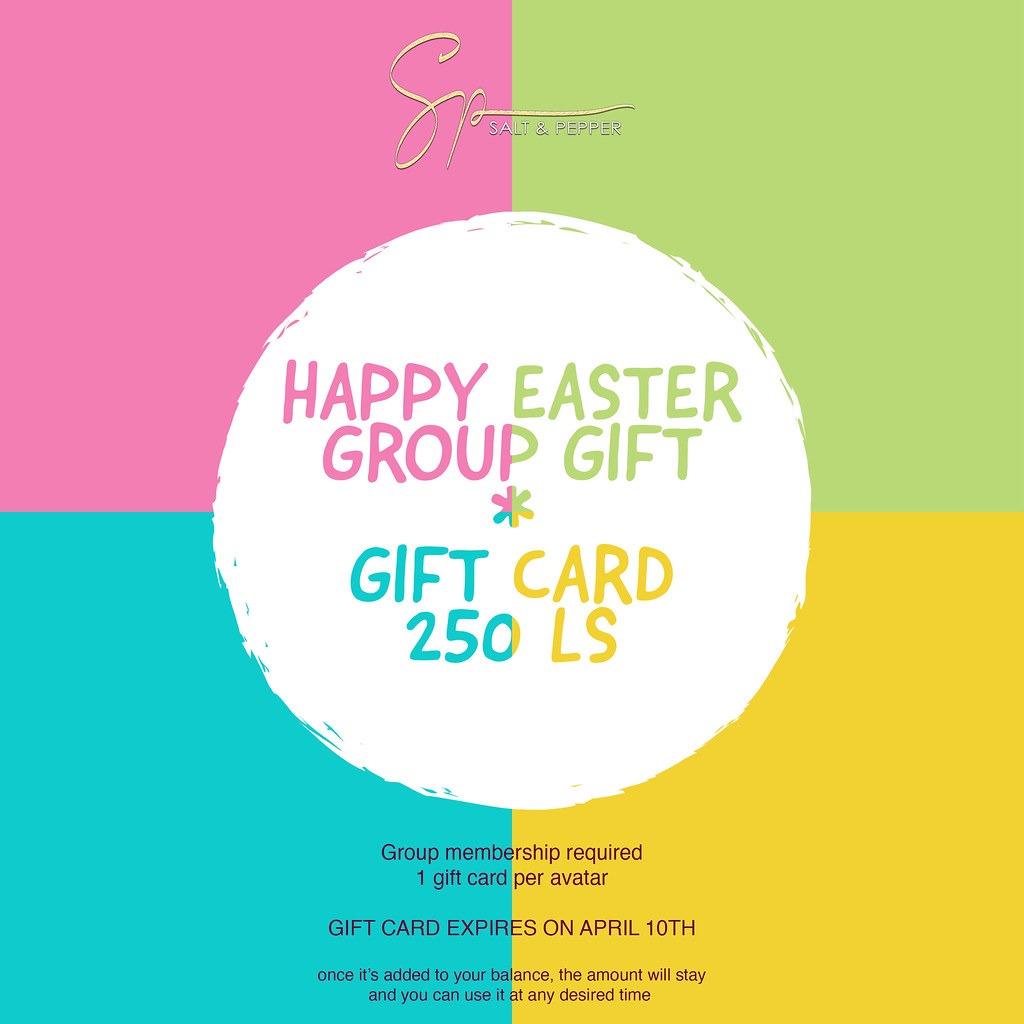The image depicts a colorful gift card advertisement designed in a square format with four distinct colored quadrants—each in a different shade: light pinkish-purple on the upper left, sage green on the upper right, light teal blue on the lower left, and goldish yellow on the lower right. Centrally positioned within these quadrants is a white circular area. Above the circle, there is script text in lime green, reading “SP” in cursive. Below this, the text "Salt and Pepper" appears in red and yellow font. Inside the circle, prominent text announces "Happy Easter Group Gift" with a small star symbol, and "Gift Card 250 LS." At the bottom of the circle, smaller text details the group membership requirement, stating "Group Membership Required, One Gift Card Per Avatar. Gift Card expires on April 10th. Once it is added to your balance, the amount will stay, and you can use it at any desired time." The overall design integrates these elements into a vibrant, multi-colored advertisement promoting a special Easter-themed group gift card.